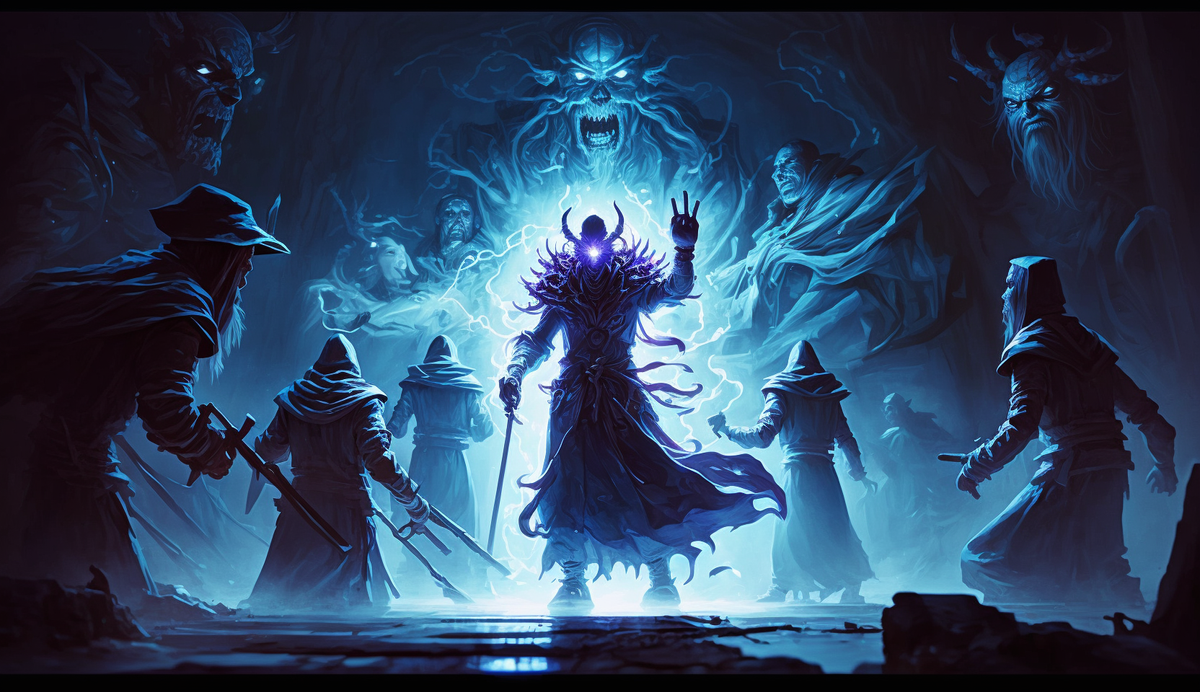In a vivid, predominantly blue and black computer-generated image, a central horned figure, akin to a wizard or demon, commands the viewer's attention. This character possesses a terrifying blend of monstrous traits, including serpentine forms slithering from his shoulders and torso, and a menacing demeanor marked by sharp teeth and a screaming, demonic expression above his head. 

Enveloped in an intense purple glow and backed by striking lightning bolts, the figure raises his right hand, displaying three fingers, while gripping a sword. His head is illuminated with a brilliant white-purple light, creating a stark contrast against the dark, shadowy background where more demonic entities lurk, their sinister visages leering from both the left and right sides.

On the reflective ground beneath this fearsome scene, several draped figures, reminiscent of monks or druids, advance cautiously towards the central figure, weapons in hand. These foreground figures, alongside a backdrop of various other fantasy creatures, all seem drawn to the ominous figure’s potent aura. The entire image is suffused with a cool blue tint, adding to the eerie, otherworldly ambiance, and is framed from a low vantage point, accentuating the imposing presence of the central character.